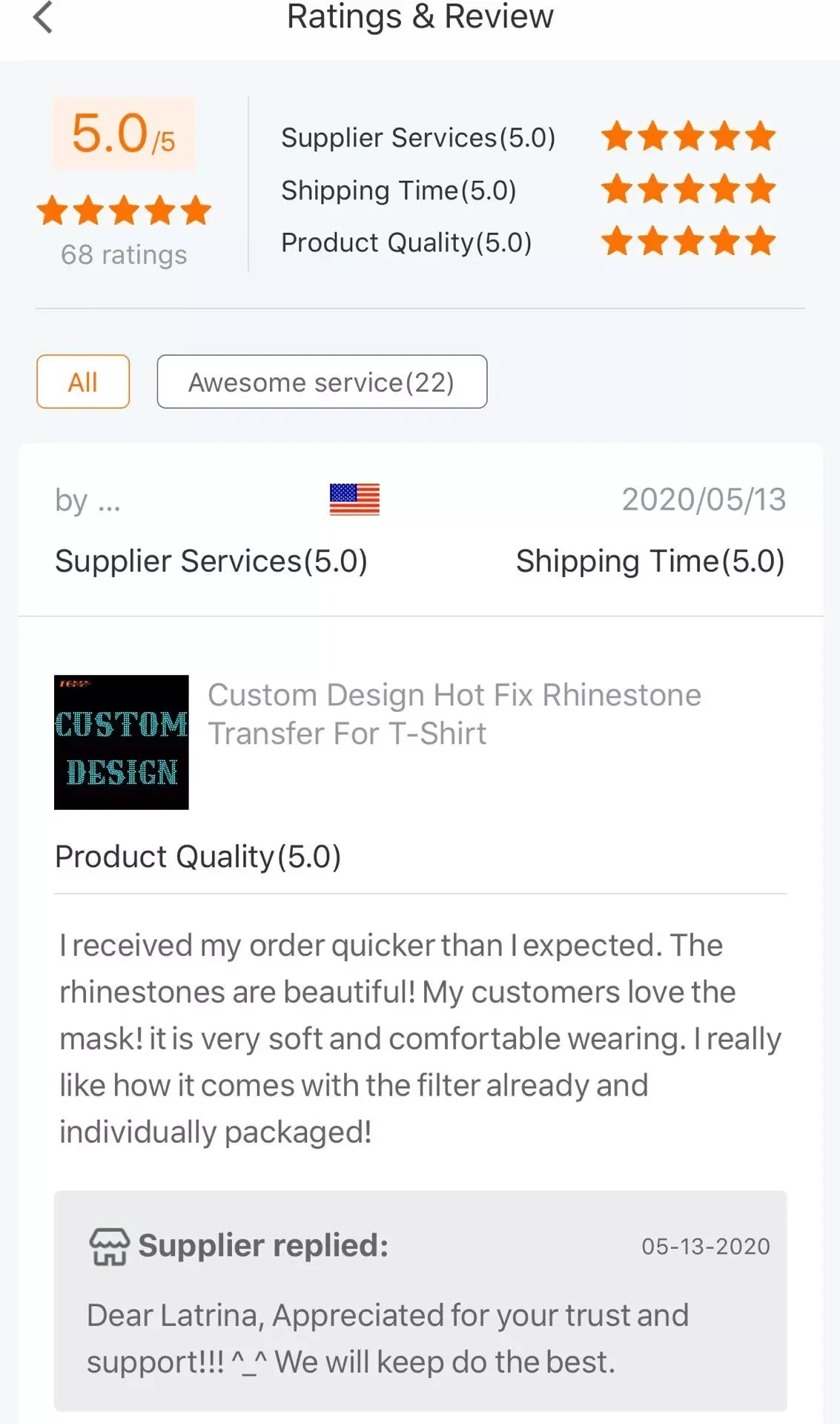**Screenshot of Ratings and Reviews for a Supplier**

At the top of the image, a back arrow icon is displayed, with "Ratings and Reviews" prominently centered. Below this heading, the supplier's overall rating is shown as an impressive 5.0 out of 5 stars, based on 68 ratings. The detailed breakdown reveals perfect scores in all categories: Supplier Services (5.0), Shipping Time (5.0), and Product Quality (5.0), with 5-star ratings for each.

The background is a subtle light grey, providing contrast for the black text. Below the ratings summary, a thin horizontal line separates this section from interactive elements. An outlined button in orange contains the word "All" in matching orange text, likely a filter option for viewing all ratings. Adjacent to it, an orange-tagged button highlights a specific review aspect tagged "Awesome Service" with 22 related ratings.

Beneath this section, a review is partially visible. The reviewer's tag features an American flag, indicating location. Their rating details follow: Supplier Services (5.0), Shipping Time (5.0), dated 2020-05-13. The review mentions "custom design, hotfix, rhinestone transfer for t-shirt," with Product Quality rated at 5.0. The reviewer praises the speed of delivery, the quality of the rhinestones, and the appeal to their customers, specifically mentioning masks' softness, comfort, and included filters packaged individually.

Additionally, a grey rectangle contains a supplier's reply, dated 05-15-2020, addressed to "Dear Latrina." The supplier expresses appreciation for the reviewer's trust and support and commits to maintaining their high standards: "We will keep due the best."